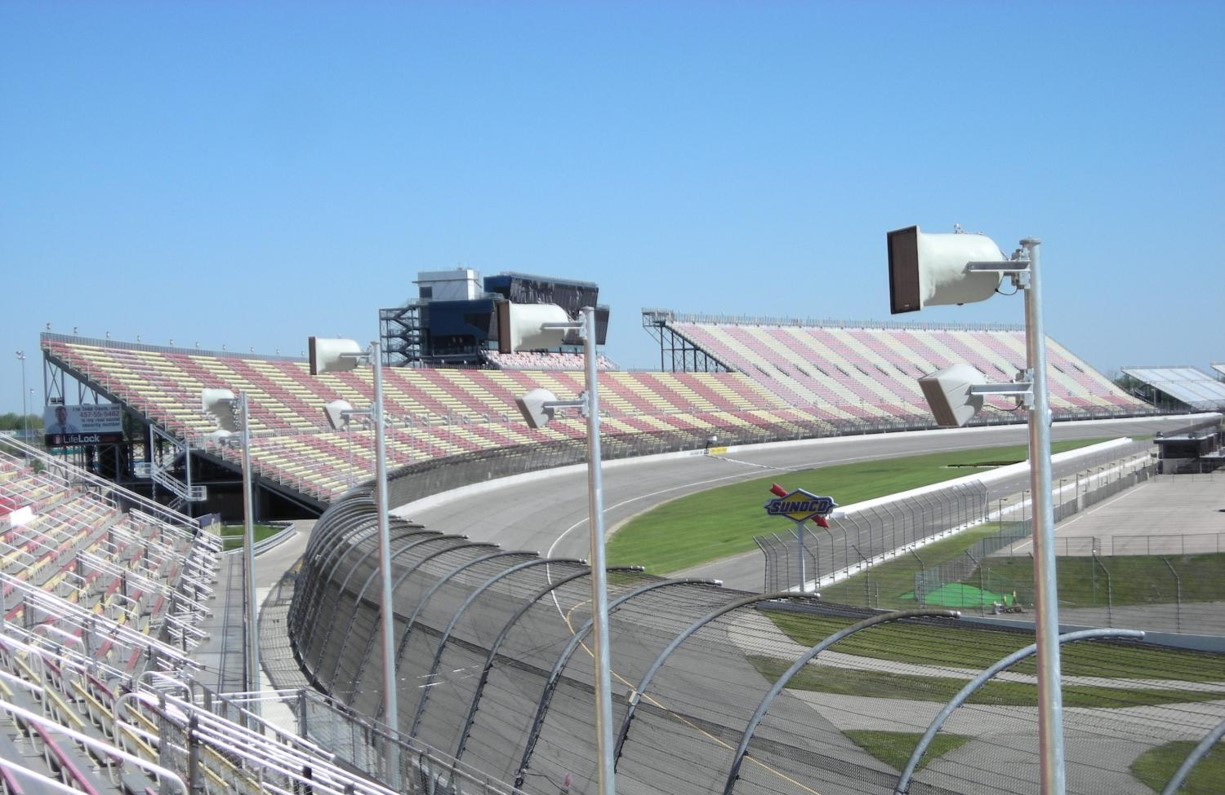This high-angle photograph from the Michigan International Speedway captures the sprawling, empty stands on a sunny day with a bright blue sky overhead. The image showcases the vastness of the speedway with its neatly mowed green grass and the alternating red and yellow striped seating. The racetrack curves prominently in the foreground, indicating its position near the first turn from the starting line. A Sunoco Petroleum advertisement sign in yellow, white, and blue stands out against the clear backdrop. High above the bleachers, loudspeakers and the judges' and statisticians' stands are visible, poised for action. Despite the absence of people and cars, the scene exudes readiness for a race, accentuated by the natural daylight illuminating the entire setting.